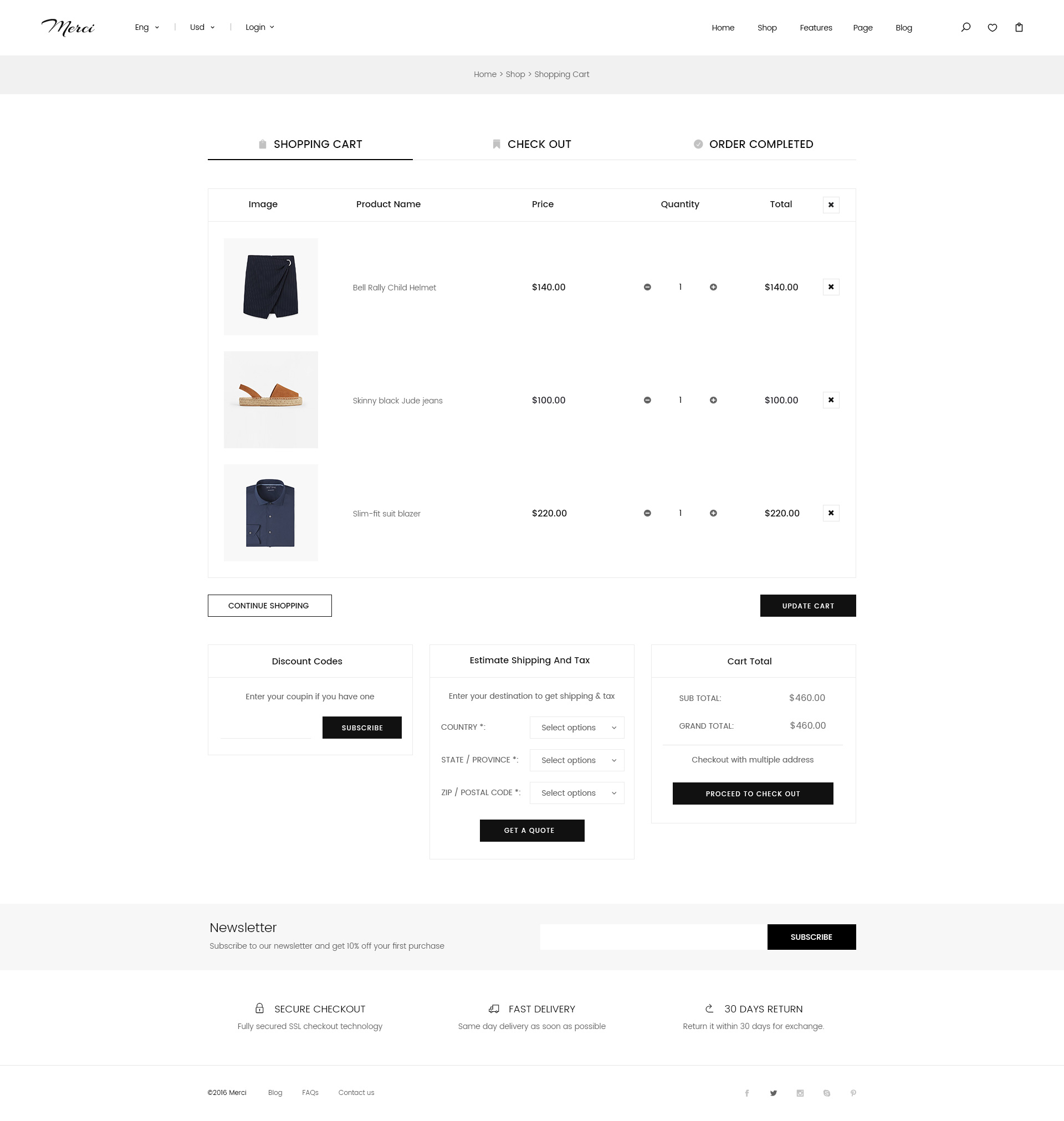Here is the cleaned-up and detailed caption:

---

This image is a screenshot of a clothing website named "Merci," elegantly displayed in cursive at the top left corner of the page. Positioned to the right of the site name, there are three dropdown menus labeled "ENG" for the language selection set to English, "USD" for the currency selector, and a "Login" option. 

At the top right, a navigation bar features five buttons: "Home," "Shop," "Features," "Page," and "Blog." Adjacent to these, icons for search (a magnifying glass), favorites (a heart), and downloads/sharing (a drop box-like symbol) are also visible.

Beneath this main navigation, a gray bar indicates the user's current location on the site, showing a breadcrumb trail: "Home," "Shop," leading to "Shopping Cart." The cart contains three items: a "Bell Rollie Child Helmet" priced at $140, "Skinny Black Jude Jeans" for $100, and a "Slim Fit Suit Blazer" costing $220.